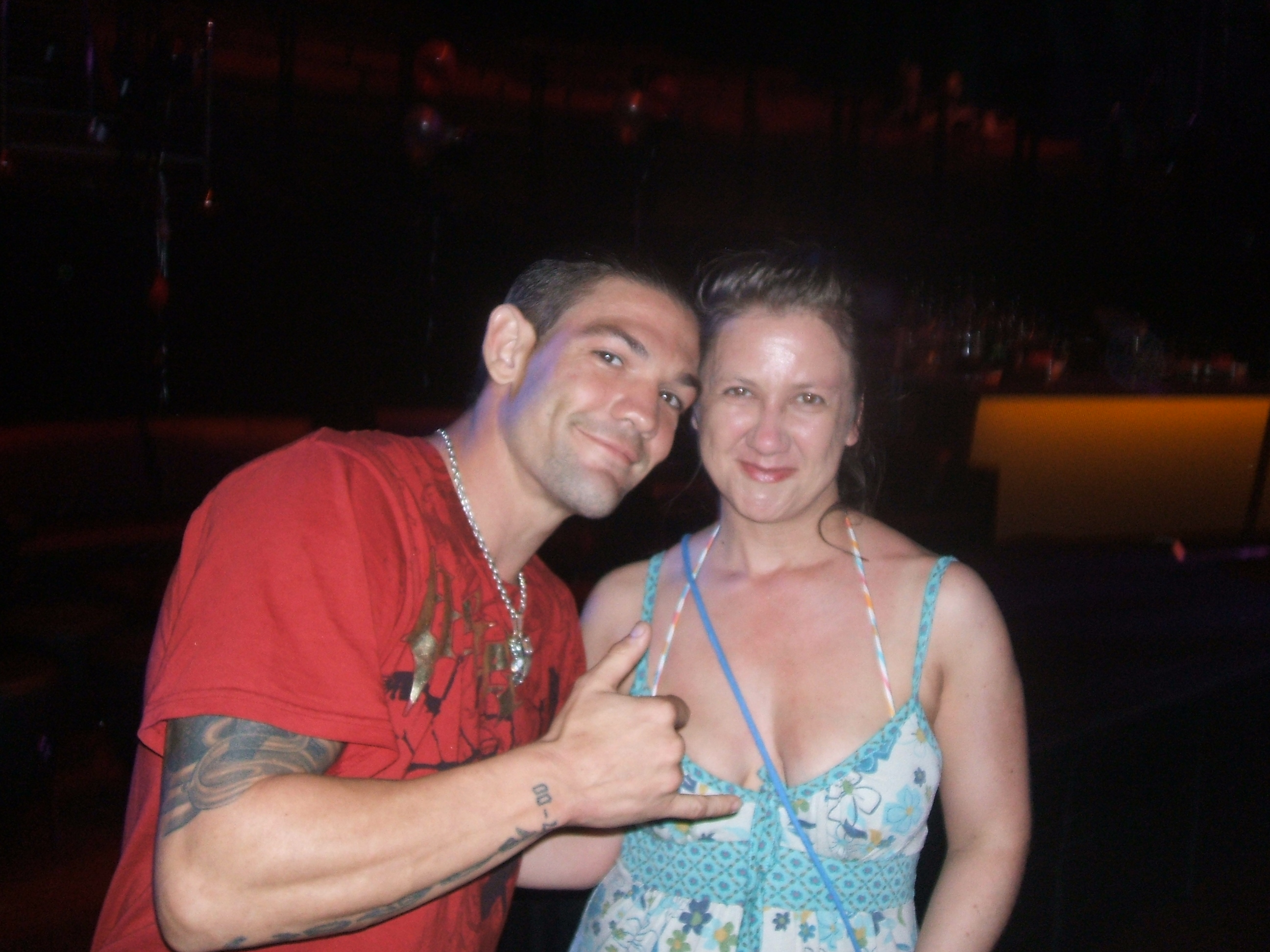This wide rectangular photograph features a man and a woman posing together in what appears to be a dimly lit bar. The background is predominantly dark and blurry, with some indistinct shadows and what looks like a bar with glasses visible on the right side of the image. The man, positioned on the left, has white skin and short brown hair, and his head is tilted slightly towards the top right corner. He has dark, raised eyebrows and a closed-mouth smile while looking directly at the camera. He wears a red T-shirt adorned with a black and gold design and a silver necklace. His arm, which is tattooed, is bent, making a hang loose sign with his thumb and pinky extended.

Next to him on the right is a woman with white skin and short blonde hair, also smiling and looking at the camera. She wears a colorful ensemble, including a rainbow bikini partially covered by a teal tank top featuring an array of turquoise, blue, dark blue, white, and yellow floral patterns. The overall scene suggests they might be in a deserted bar with the lights turned off, yet both are well-lit and appear happy and content.